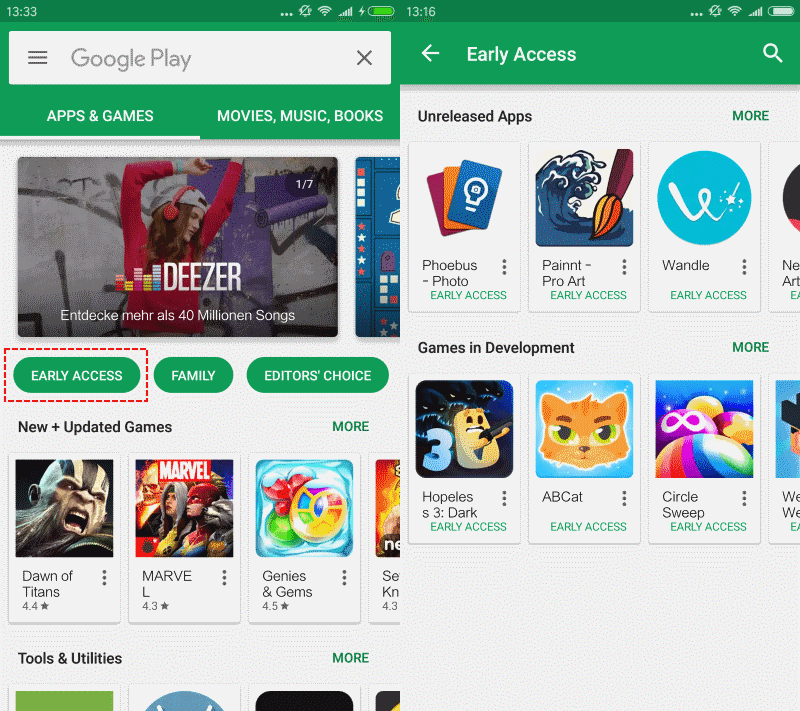The image consists of two side-by-side screenshots from the Google Play Store. 

On the left side, the screenshot displays the main search interface for apps and games, characterized by a prominent white and green search bar at the top. Elements of the broader navigation options such as movies, music, and books are visible but not focal to the current search results. Below the search bar, the screen showcases a selection primarily featuring games. Notable titles listed under "New and Updated Games" include "Dawn of Titans," "Marvel," and "Genies and Gems," among others. Positioned further down the page, although partially cut off, are categories for tools and utilities. The screenshot has been annotated with a dashed box highlighting the "Early Access" tag, signifying new and in-development apps and games that users can explore.

On the right side, the screenshot focuses on the "Early Access" section explicitly. It is labeled as a collection of unreleased apps and games that are currently in development, allowing users early access to try them. Featured unreleased apps include "Phoebus Photo," "Paint ProArt," and "Wondle." In the realm of in-development games, the titles "Hopeless 3," "ABCat," and "Circle Sweep" appear, which seem targeted towards a younger audience.